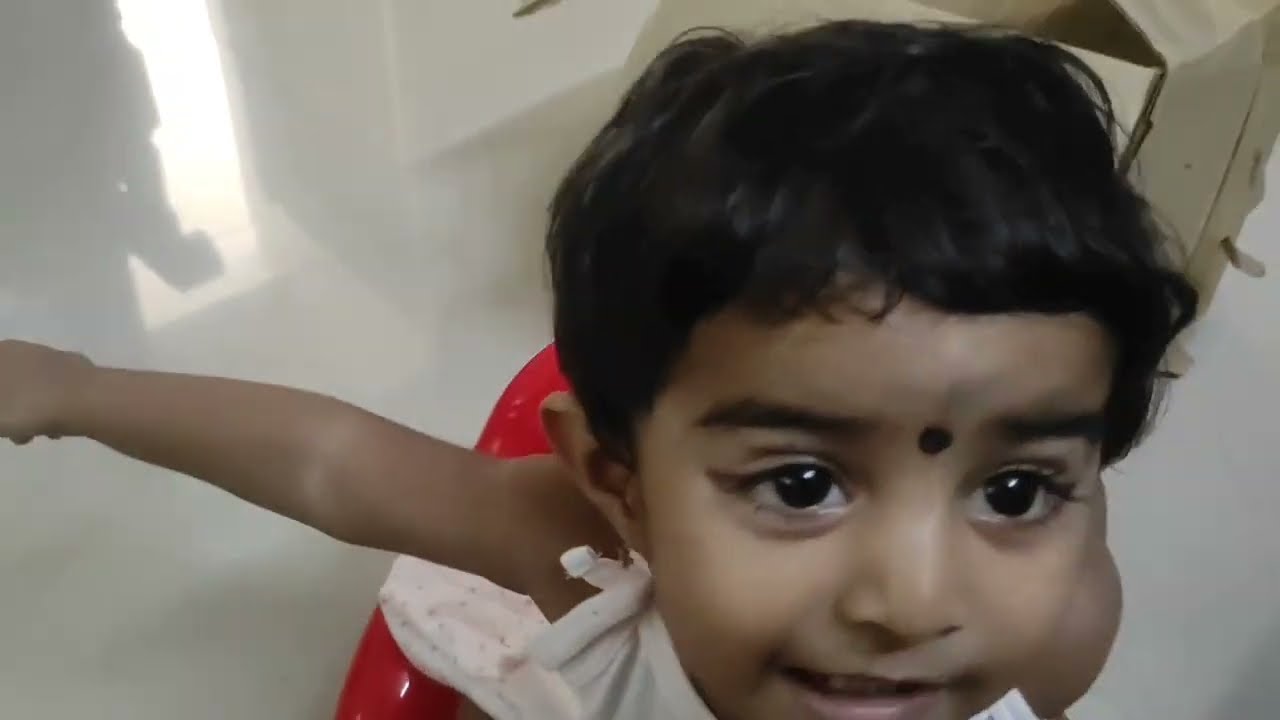This photograph features an up-close image of a young Southeast Asian child, approximately two to three years old, with short, dark brown hair and very short bangs, accompanied by a small black dot between their eyebrows at the top of their nose. The child has large brown eyes and is looking slightly off to the side with a subtle, happy smile. They are wearing a white top and a red skirt, though only a small sliver of the outfit is visible on the left-hand side. The child has one arm fully extended outwards. In the background, the floor and walls are stark white, and the back left-hand corner shows a vague black shadow, possibly a person or another object. Additionally, a beige-colored cardboard box is noticeable in the upper right corner. The image appears to be a personal indoor photo, likely taken in the middle of the day, with the child positioned centrally on what might be a shiny, red cushion or chair.